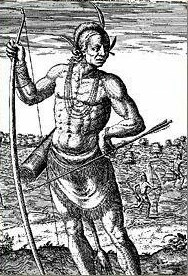The image is a meticulously detailed, old etching from what appears to be the 1700s, rendered entirely in black and white. It depicts a Native American warrior prominently positioned in the foreground, holding a very tall, simple longbow in his right hand, and an arrow in his left hand, poised as if he is preparing to shoot. The bow is so large that it is taller than he is. He is adorned with several feathered embellishments in his hair, which is styled in a braid. The warrior’s attire consists of a simple loincloth skirt, leaving his upper body and legs uncovered, and he is accessorized with four rows of beaded necklaces. There is a quiver of arrows slung across his back, hanging off to his side. The background is intricately busy with sky and clouds at the top, though the finer details are hard to make out. In addition, there appears to be faint images of two figures in the background, potentially indicating a hunting scene. The etching is highly detailed with shading done likely in pen or pencil, reminiscent of illustrations found in historical books or encyclopedias.